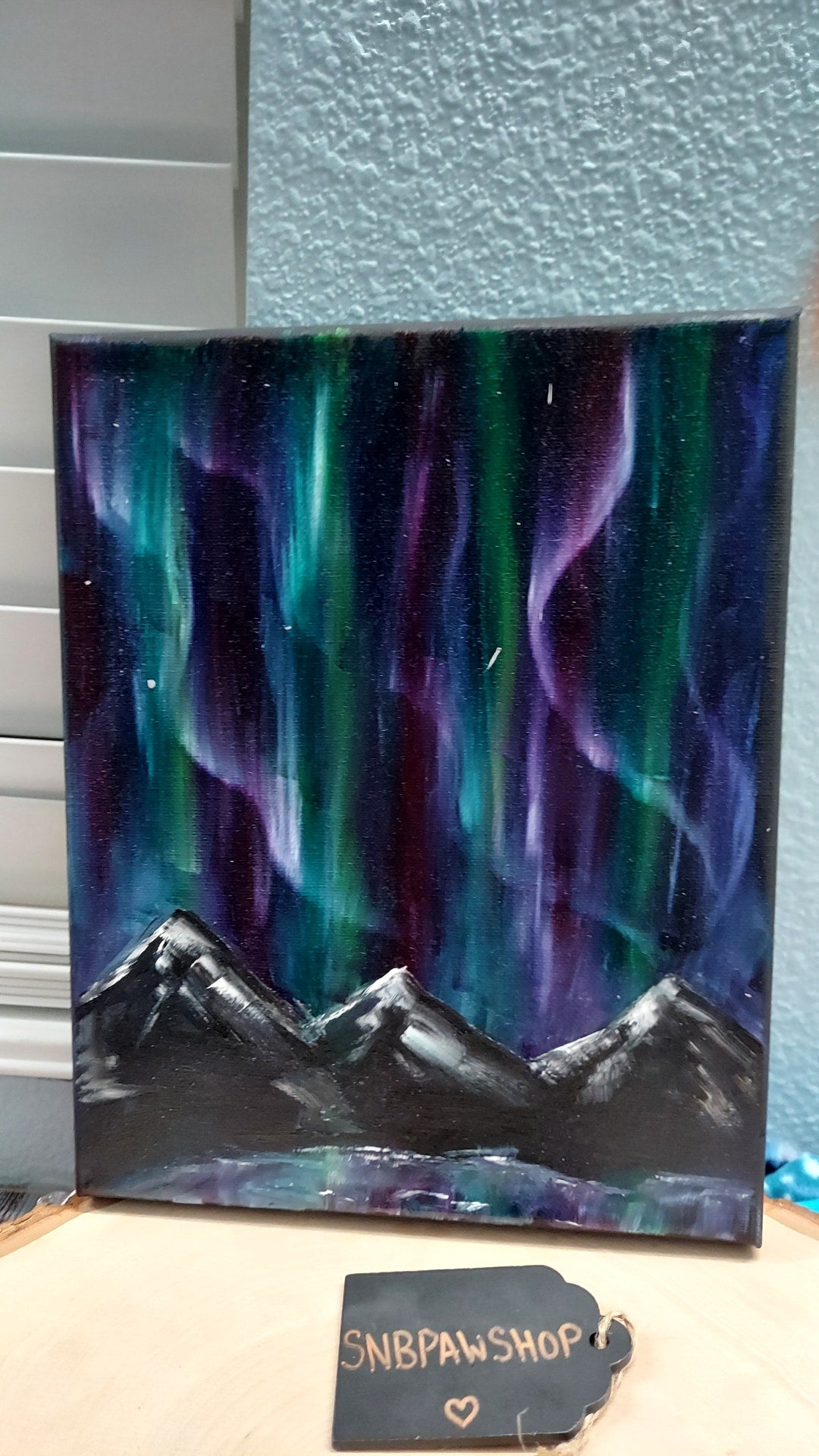This is a color photograph of a handmade painting depicting the Aurora Borealis, or Northern Lights, resting on a light pink surface. The painting features three mountain peaks lightly dusted with snow and portrayed in shades of black, gray, and white. Above the mountains, vibrant waves of Northern Lights dance across the night sky in hues of bright green, purple, and blue, creating a ghostly, mesmerizing effect. At the base of the painting is a reflective body of water mirroring the colorful Aurora.

The painting is propped against a light blue, textured wall seen on the right and top edges of the image, with white mini blinds partially visible to the left side. The background includes a bit of vinyl wall as well. In the foreground, on the light pink surface, there is a black tag with gold lettering that reads "S. and B. Pawn Shop," adorned with a small heart beneath the text. The edges of the photograph also hint at a wooden table made from a tree stump, adding to the rustic charm of the scene.